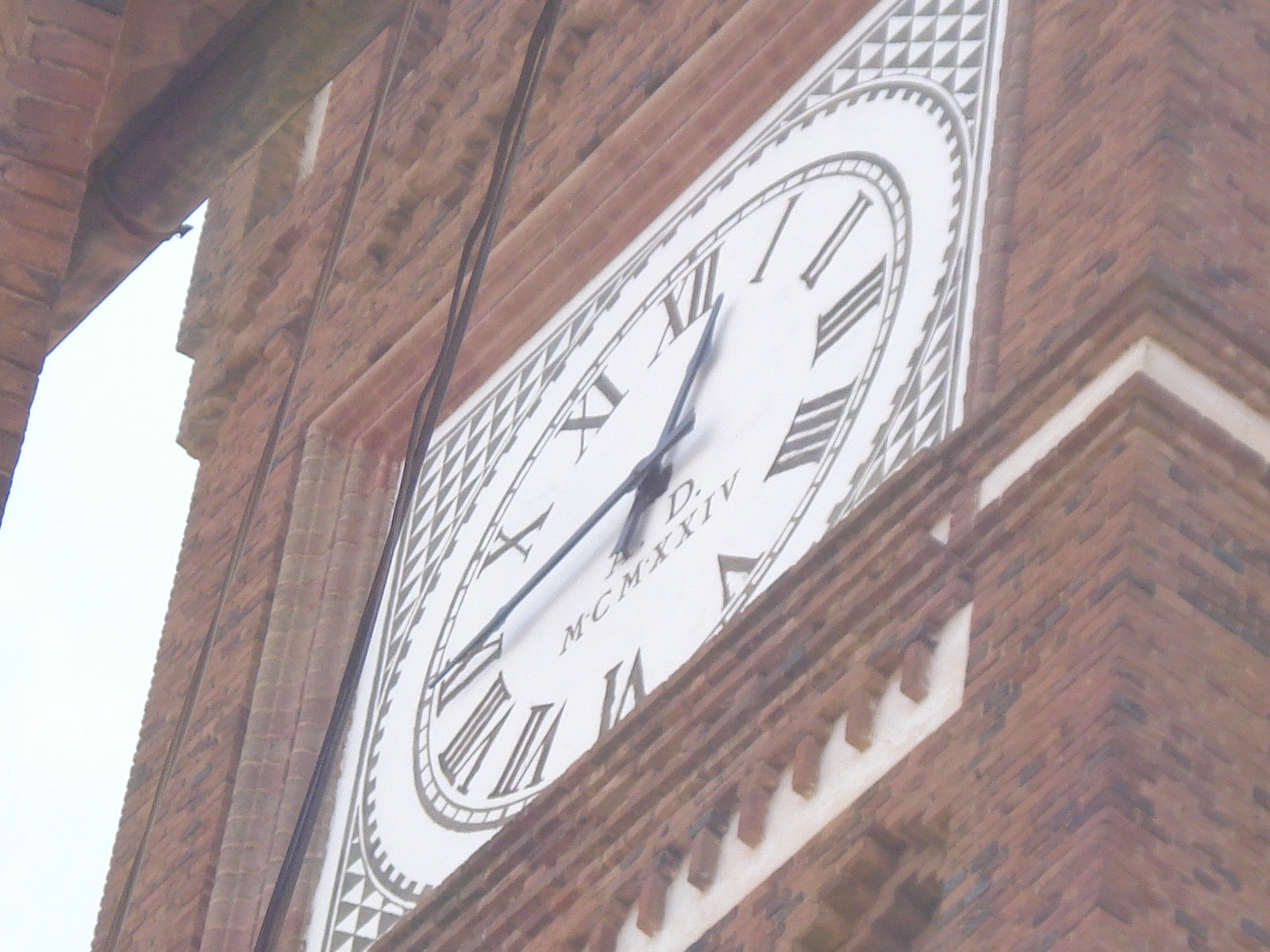Close-up of a brick tower showcasing its intricate architecture. The tower is constructed from a blend of red and brown bricks, giving it a timeless, rustic appearance. Prominently featured is a square clock face embedded in the tower. The clock’s design contrasts sharply with the brickwork, displaying a white and grey color scheme. Roman numerals from I to XII mark the clock's hours, and its hands indicate that the current time is quarter to one.